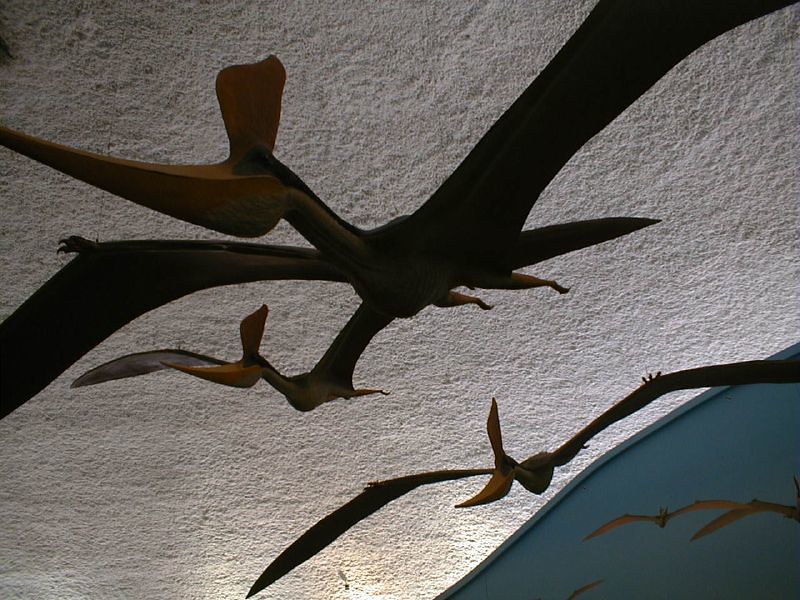This detailed photograph, likely taken in a museum, showcases a striking display of large, flying bird-like creatures. The central focus is on three prominent specimens that appear to be crafted from plaster or rubber, suspended from the textured white ceiling by thin black strings. These creatures bear a striking resemblance to pterodactyls, with elongated wings featuring hand-like claws and large, pelican-like yellow beaks topped with pronounced crests. The background includes a vivid mural of a blue sky, adding depth to the display by depicting additional birds in flight. To the lower right, smaller versions of these creatures can be seen, enhancing the impression of a dynamic, immersive exhibit. The colors are predominantly brown for the creatures, against a white and blue backdrop, emphasizing the lifelike appearance of these prehistoric-looking birds in this meticulously designed museum exhibition.